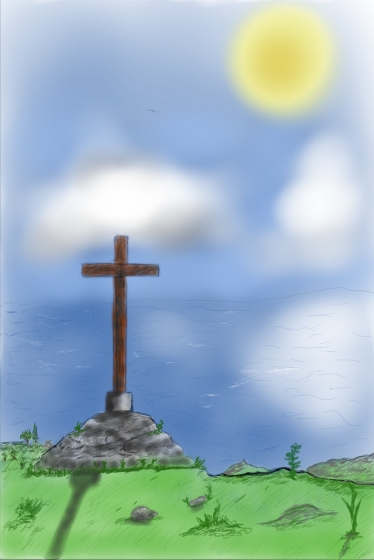This detailed drawing captures a serene landscape where a simple brown wooden cross stands slightly off-center to the left, firmly planted on a mound of grayish dirt. In the foreground, lush green grass grows vibrantly, accompanied by small plants and a tiny snail, each element meticulously illustrated. The scene extends towards a cliff or hill that drops off into an expansive sea, creating a picturesque contrast. The water below reflects the bright yellow Sun positioned in the top right corner of the image, casting a lighter patch upon its surface. The sky above is a gradient of blues, transitioning from the deeper hues of the sea to the lighter shades of the heavens, dotted with soft, blurry clouds. Though the Sun appears out of focus, adding a dreamlike quality, the entire composition conveys a tranquil and sunny day by the coast.